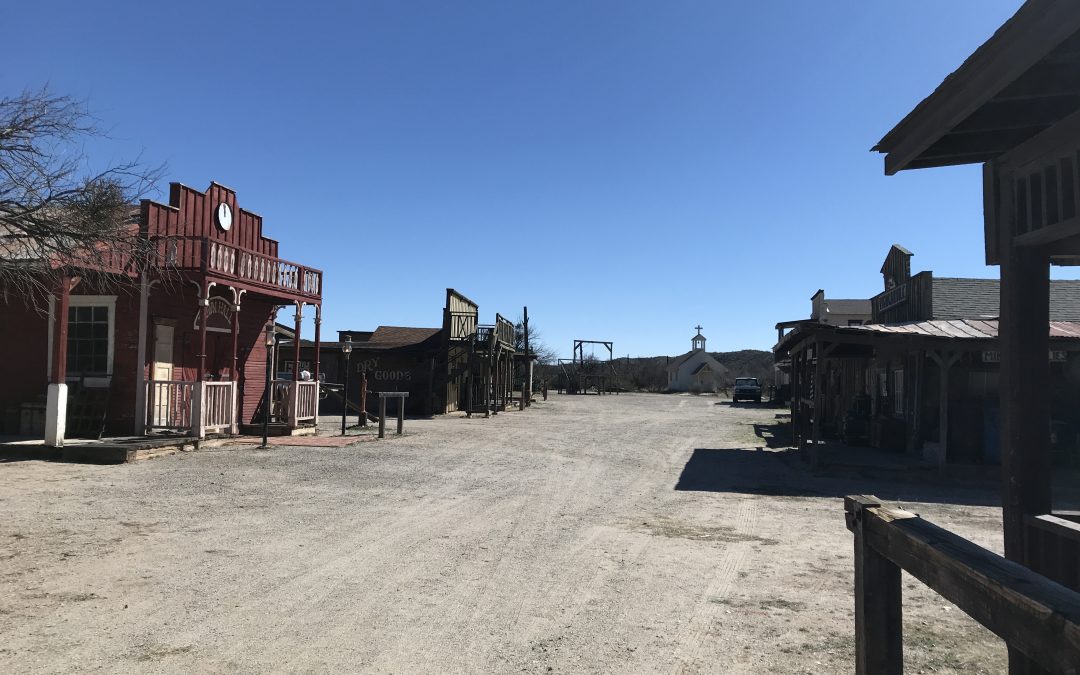This vibrant color photo captures a seemingly abandoned Wild West-style frontier town under a bright blue sky. The town, reminiscent of scenes from classic shows like "Gunsmoke" or "Bonanza," features a wide, central dirt track road that leads the eye straight down to a small white wood-paneled church with a wooden steeple and a cross on top. Several well-preserved buildings line the road. On the left, a striking auburn-colored saloon with a small porch or veranda and a clock on the second-floor balcony stands prominently. Next to it is a building marked "dry goods." On the right side of the street, shaded by the sun, there are additional dark wooden buildings, including a barbershop indicated by a traditional spinning pole and an older white truck facing the camera. Further down the road, wooden gallows are visible, contributing to the evocative ghost town atmosphere. The scene is devoid of people, enhancing its deserted and historic charm.